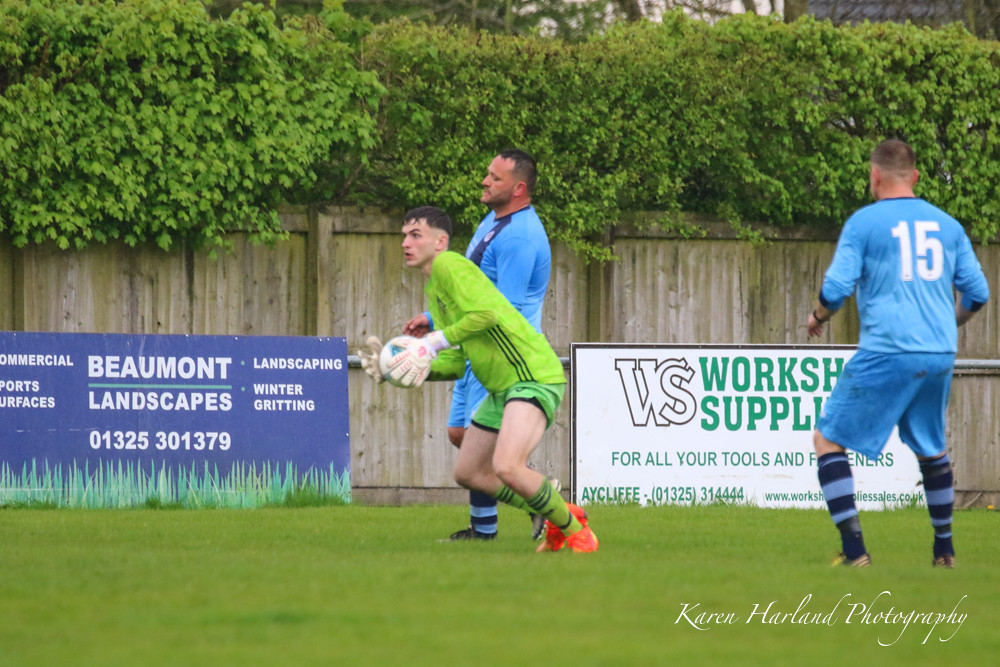The photograph captures an intense moment during a daytime soccer game on a vibrant green grass field. At the center is a goalkeeper, identifiable by his green jersey with black vertical stripes, green shorts, green socks with black trims, and orange cleats. He is seen with the soccer ball in his hands, possibly having just made a save, while slightly bent down and looking to the left. The goalkeeper's side profile shows he has short black hair and likely Caucasian features.

Behind the goalkeeper, there is another player who appears to be either challenging him or from the opposing team. This player is wearing a light blue jersey, light blue shorts, and socks that are a mix of dark blue and light blue, with black cleats. He too has short black hair and a side profile facing the left.

To the right side of the image stands another player from the blue team. His back is turned towards the camera, displaying the number 15 on his blue jersey. He is also dressed in blue shorts and socks similar to his teammate, with dark blue and light blue stripes, and black cleats. This player, who also has short black hair, is slightly obscuring a billboard in the background.

The soccer field, lush and green, is enclosed by a wooden fence topped with overgrown green bushes that stretch across the entire background. Two prominent advertisements are displayed on this fence. To the left is a horizontal sign for "Commercial Sports Surfaces" in white text on a dark blue background. Just right of this is another dark blue sign reading "Beaumont Landscapes, 01-325-301-379." Further to the right is a partially obscured white sign with green text for "Workshop Supplies for all your tools and fasteners," featuring a WS logo, a contact number "01-325-3144-44," and an obscured website. The bottom right corner of the image discreetly bears the signature "Karen Harland Photography" in cursive white font.